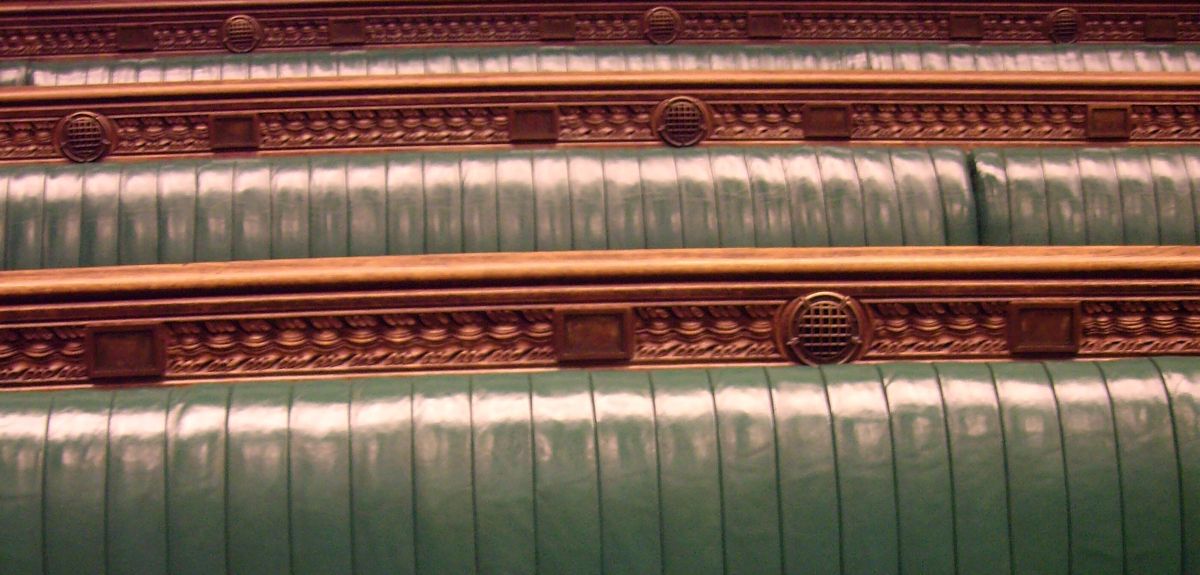The image showcases a series of rows that appear to be seating arrangements, likely in an auditorium or a church. The seating features blue or possibly dark mint green cushions, adding a color contrast to the scene. These rows of seats are accompanied by ornately carved wooden railings. The railings are brown and feature intricate round wooden carvings, adding an elegant touch to the decor. The perspective of the image shows seating in the foreground, middle ground, and background, giving a sense of depth. The wooden banisters repeat with each row, adorned with decorative buttons or carvings that enhance the overall intricate woodwork. Each row is meticulously crafted, emphasizing a harmonious blend of plush cushioning and sophisticated wooden elements.